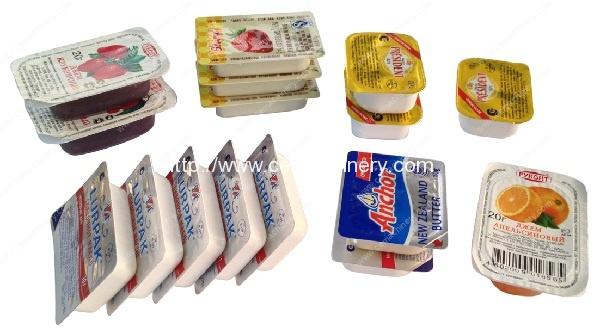The image displays an assortment of small, individual packages of spreads typically found in hotels, arranged against a white background. The packages include butters and jams, recognizable by their familiar brands and colorful labels. In the upper left section, there are packets of strawberry jam, distinguished by their white tops adorned with strawberry images and dark red plastic bases. To the right, another set of strawberry jam packets feature yellow and white stickers with strawberry graphics. Adjacent to these are three stacked packages of President Butter, marked by their yellow tops, red text, and red banners. Below, on the bottom row, the packages have a more square shape, with a silver top and blue text on the leftmost one, indicating Lubrak butter. Next to it is a packet labeled Anchor in red text, identifying it as another butter variety. The bottom-right corner of the image reveals a package of orange jam, completing the array of breakfast spreads.